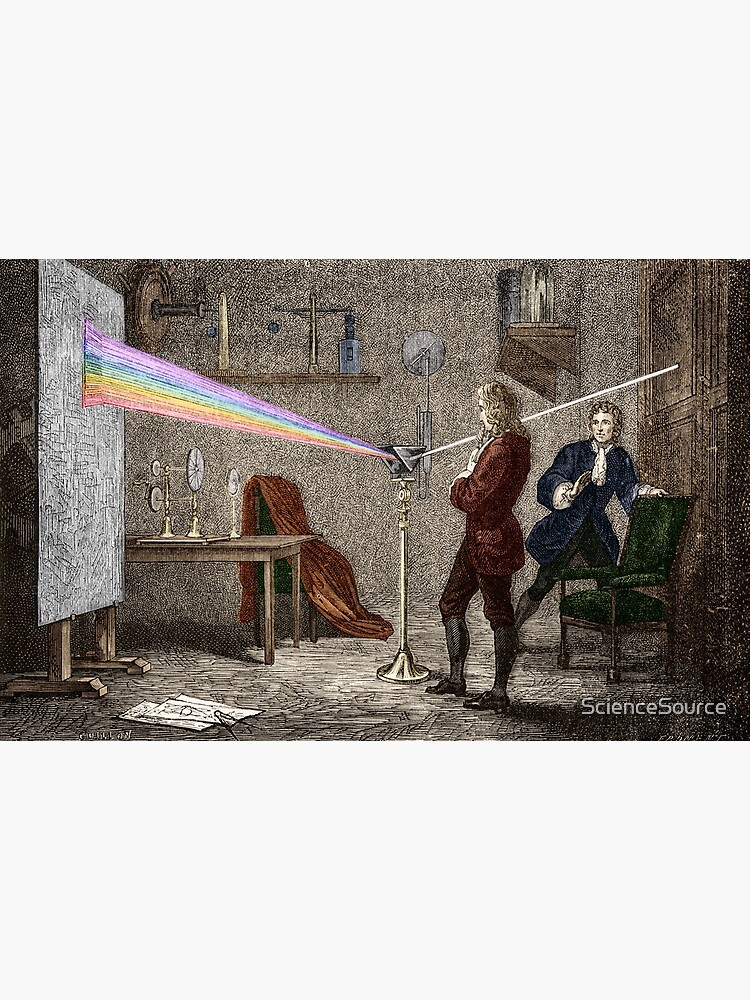The image is a detailed indoor illustration of a scientific experiment from the 18th century. In the center of the room stands a man dressed in period attire—long pants, gray boots, a brown shirt, and boasting long, blondish hair. He is intently observing a device, a stand holding a prism, situated in the middle of the room. A beam of white sunlight enters from a small opening on the right side of the room, striking the prism and dispersing into a spectrum of rainbow colors—red, orange, yellow, green, blue, indigo, and violet—that are projected onto a gray screen set up on the left side of the room.

Behind the central figure, there is a younger man with shorter hair, wearing a black jacket that spreads out like a skirt along with leggings and boots. This man, looking somewhat surprised, stands with his hand on a chair. The room is furnished with a desk, chairs, shelves holding various scientific instruments, including one shaped like a cross, and a table next to the screen with additional equipment on it. There is also a noticeable watermark at the bottom right-hand corner that reads "Science Source."

This illustration seems to depict Isaac Newton's experiment demonstrating the refraction of light using a prism, revealing how light is composed of different colors.